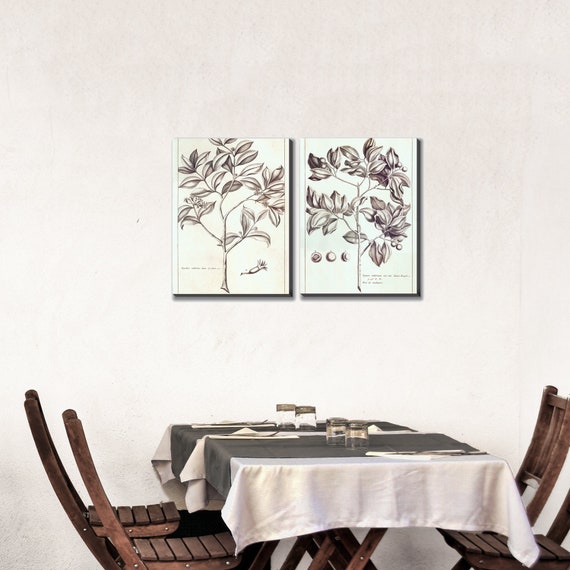The color photograph features a dining table set meticulously for four people. The table, crafted from rich dark wood, is adorned with a pristine white tablecloth and a gray overlay. Two sets of two drinking glasses are strategically placed upside down on the table, accompanied by neatly folded white napkins and silverware laid atop them. The scene exudes elegance with four brown wooden chairs, positioned with two on each side of the rectangular table. The dining setup is set against a simplistic white wall, which is accentuated by two centered artworks above the table. These ink drawings on white canvas depict the graceful, curvilinear form of plant leaves, rendered in natural and elegant lines. The overall ambiance is one of understated sophistication and careful attention to detail.